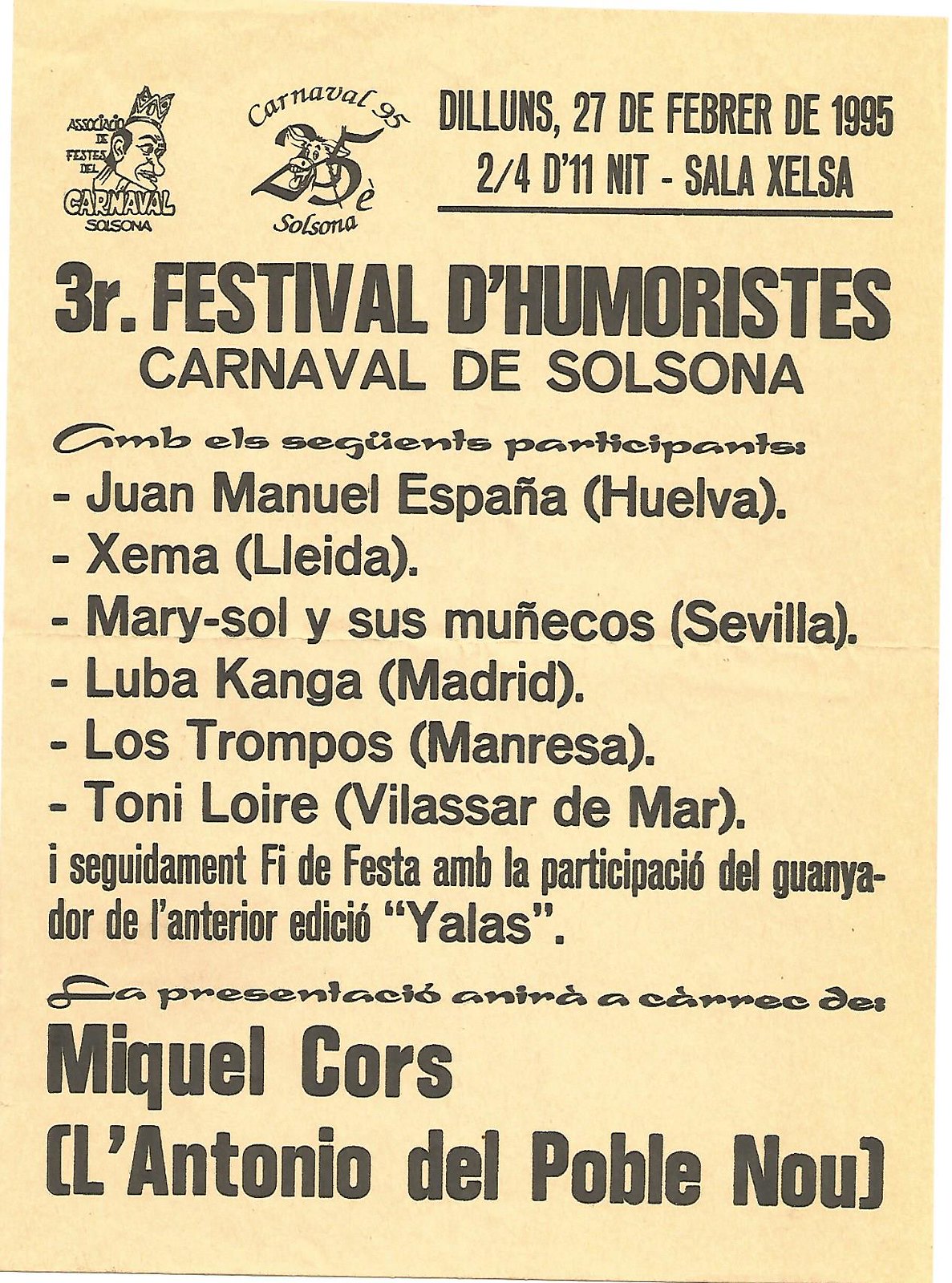The image is a detailed poster advertising the "Third Festival of Humorists," also known as "Carnaval de Solsona." The poster is printed in black ink on beige, tan, or pink paper, with all text in Spanish. On the left side of the poster, there is an image of a man’s head and neck, adorned with a crown. The prominent text includes the phrases "Carnaval de Solsona," "3R Festival de Humoristes," and "Carnaval 95 Solsona." The event is scheduled to take place on "lunes 27 de febrero de 1995" at "Sala Excelsa." The poster lists various participants in a bulleted format, including names such as Juan Miguel España (Lleida), Marisol Isos Murcielagos (Sevilla), Lubacanga (Madrid), Los Trapos (Manresa), and Tina Maria (Llassa de Mar). At the bottom of the poster, the names Miguel Corse and Antonio del Poblenou are highlighted, each followed by their respective details within parentheses.